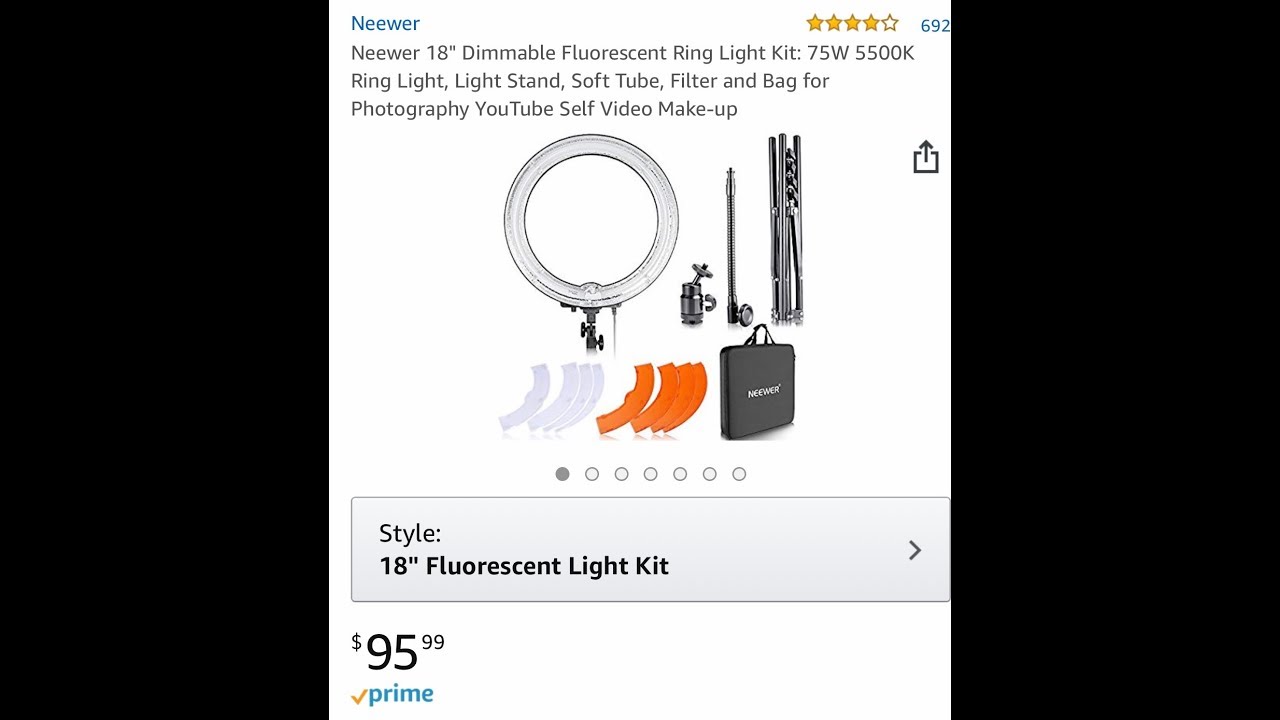Here's a detailed and cleaned-up caption for the image described:

---

The screenshot showcases a product page on Amazon for the Neewer 18-inch Fluorescent Ring Light Kit. This versatile lighting system is ideal for photography, video recording, selfies, and makeup application. The complete kit includes a 75-watt, 5500K ring light, a light stand, a soft tube, and filter options for customizable lighting. It also comes with a carrying bag for portability. The package features white and orange curved filters for different lighting effects, and three cords for setup. The product has garnered a commendable rating of 4 out of 5 stars from 692 reviews. Priced at $95.99 with Prime shipping, the page includes seven swipable images showcasing various aspects of the kit. Multiple style options are available for buyers to choose from.

---